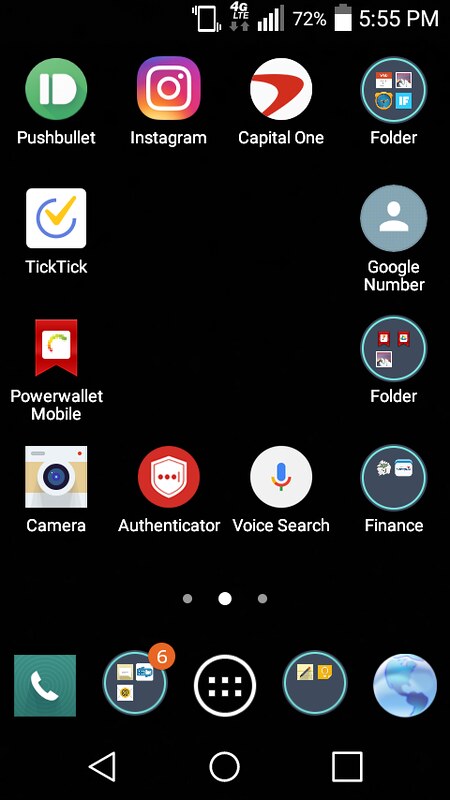The image depicts a smartphone screen showcasing various icons and widgets. At the very top left corner, there is an icon indicating the phone is in vibration mode. Next to it, the display shows a 4-bar signal strength, a battery level at 72%, and the time as 5:55 PM.

Starting from the top left, there is a Pushbullet icon, which is represented by a vertical white line and the letter "D" inside a green circle. Adjacent to this is the Instagram symbol. Next is the Capital One app icon, represented by a red boomerang. Following this is a folder icon containing four sub-icons.

Continuing to the left on the second row, there is the TickTick icon characterized by a blue "C" and a checkmark. To its right is the Google Contacts app symbolized by a generic contact icon. Further right, there's the PowerWallet Mobile app, represented by a red flag with a colorful arc. On the far right, another folder icon appears, this time containing three sub-icons.

The row below features a camera icon with a minimalistic design, including a lens and a recording light indicator. Next is the Authenticator app icon, distinguished by a big red circle and a shield with dots inside it. Additionally, there is a Voice Search icon depicted as a blue microphone with red and white highlights.

At the bottom row, towards the left, a green square with a white phone icon is visible, accompanied by three additional icons. There is also a circle with six dots on the top right section.

Finally, the very bottom right features an icon of a globe with some graphical elements beside it, including shapes such as a triangle, a circle, and a square. Multiple app and folder icons are arranged around these main features, creating a comprehensive layout of the smartphone's home screen.